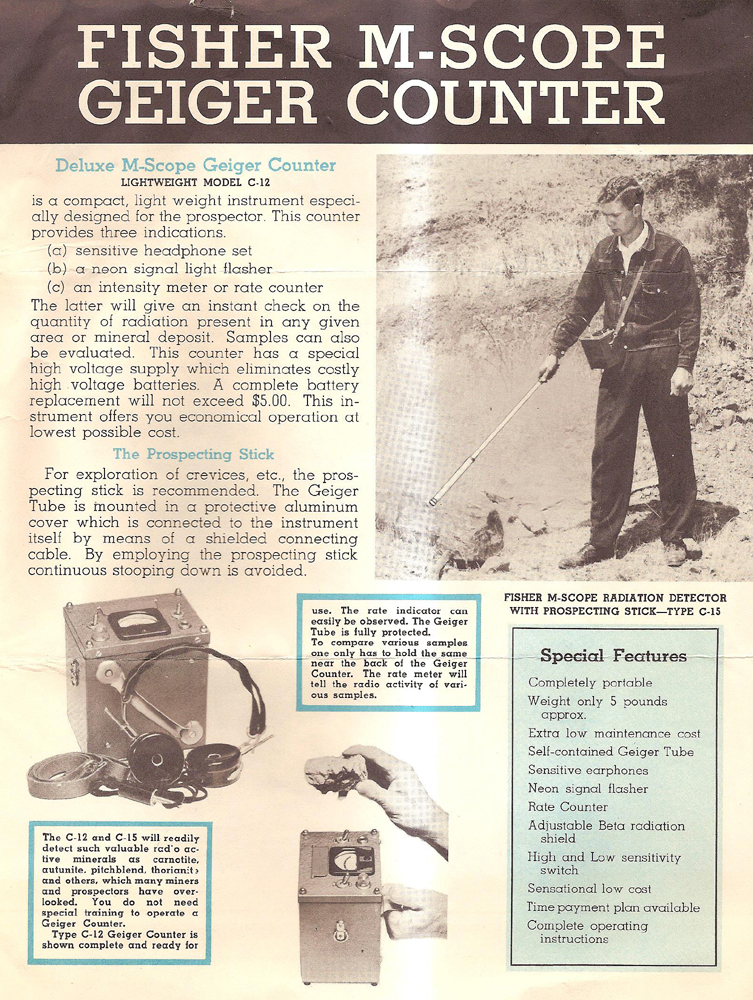This is a vintage, black-and-white advertisement for the "Fischer M-Scope Geiger Counter," most likely sourced from an old newspaper, magazine, or possibly displayed on a building wall. At the top of the ad, bold text reads "Fischer M-Scope Geiger Counter," followed by a detailed description of the "Deluxe M-Scope Geiger Counter C12 Lightweight Model." The advertisement outlines the device's features, including a sensitive headphone set, neon signal light flasher, and an intensity meter or rate counter.

To the right of this text, there's a black-and-white photograph of a young man with dark hair, dressed in plain clothes, holding a long stick as he surveys the ground with intense concentration. Attached to his shoulder by a strap is a box-like Geiger counter, suggesting he is using the device for prospecting.

Below this, another photograph shows a close-up of the Geiger counter, equipped with a pair of headphones lying next to it. Adjacent to this image, a supplementary photo captures someone's hands holding a rock and manipulating the dials on the box-like device, emphasizing the practical use of the counter in the field.

On the right-hand side of the advertisement, a blue box labeled "Special Features" lists various important specifications and capabilities of the Geiger counter, consolidating the detailed promotional pitch aimed at prospective buyers.